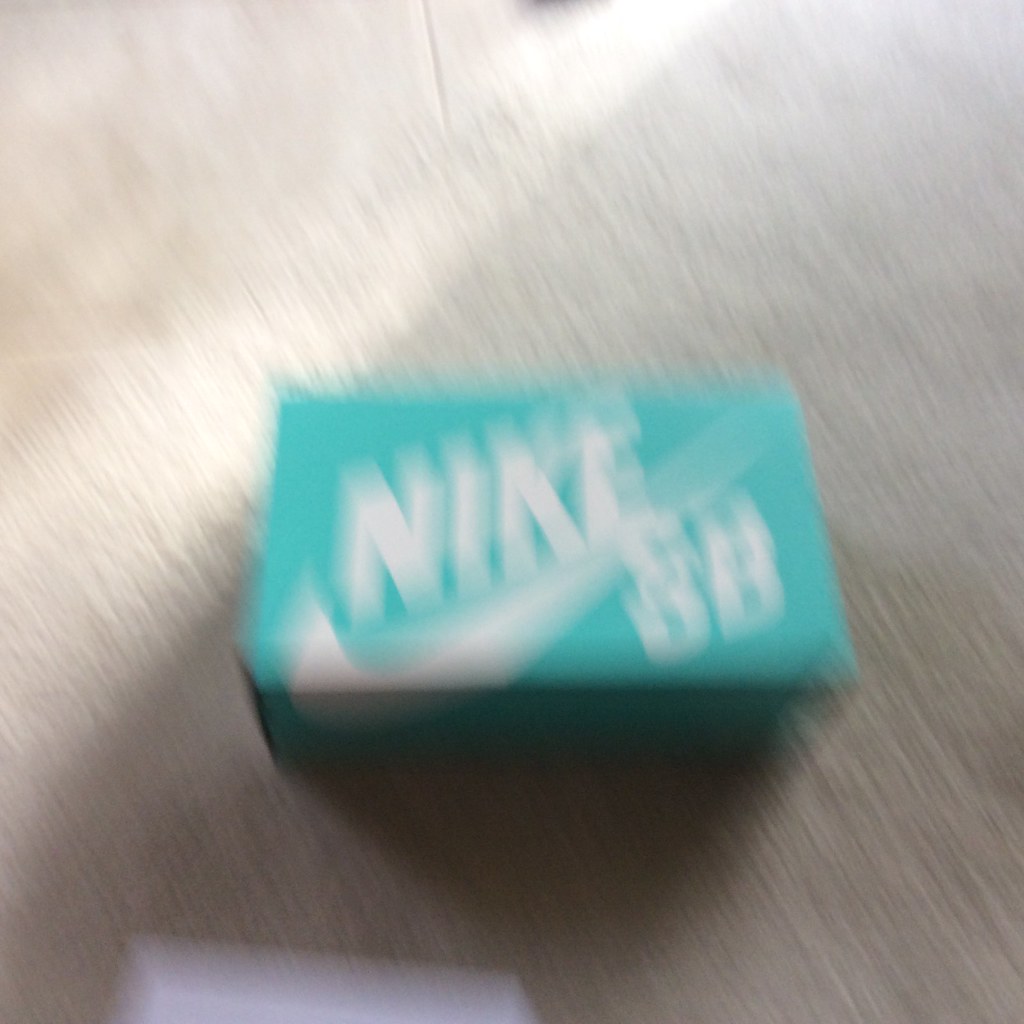The image depicts a blurred photograph of a Nike shoe box. The box features a striking aqua color that stands out despite the blurriness. Prominently displayed on the top of the box is the iconic Nike Swoosh logo in white, with the letters "SB" appearing underneath it, albeit slightly blurred. The setting appears to be a beige carpet, although the blur suggests the camera was in motion when the picture was taken. In the lower left corner, you can vaguely make out another white object, possibly another box or container. There seems to be an additional indistinguishable object at the top of the frame, adding to the scene's overall clutter. The presence of a groove in the ground and a noticeable shadow cast by an off-camera object indicates an overhead light source. The lighting suggests natural light possibly coming from a living room window. Overall, despite the lack of clarity, the image captures a snapshot of what appears to be a casual indoor setting.